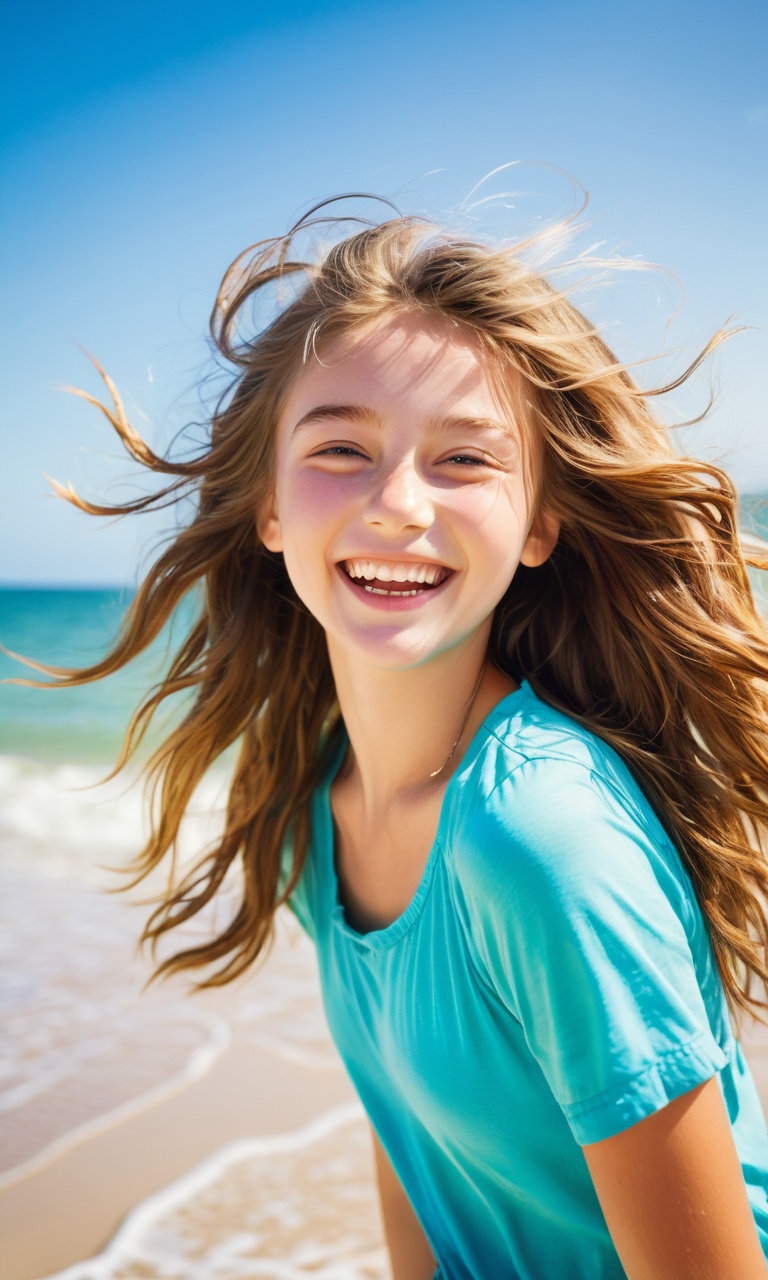A vibrant close-up image captures a smiling young girl at the beach, likely around 11 or 12 years old, with her dark blonde hair flowing in the wind. Her expressive face, featuring slightly closed eyes shielding from the bright sun, showcases a broad smile, revealing both upper and lower teeth. She is dressed in a turquoise short-sleeved T-shirt. The background displays a serene beach scene: the deep blue ocean waves are gently slapping onto the sandy shore below, while the sky transitions from a whitish cloudy hue to a deeper blue towards the top of the image. Her joyful and carefree demeanor is the focal point, with her arms resting naturally by her sides. The setting sun, positioned in the upper right, casts a warm light across the scene, enhancing the overall cheerful atmosphere.